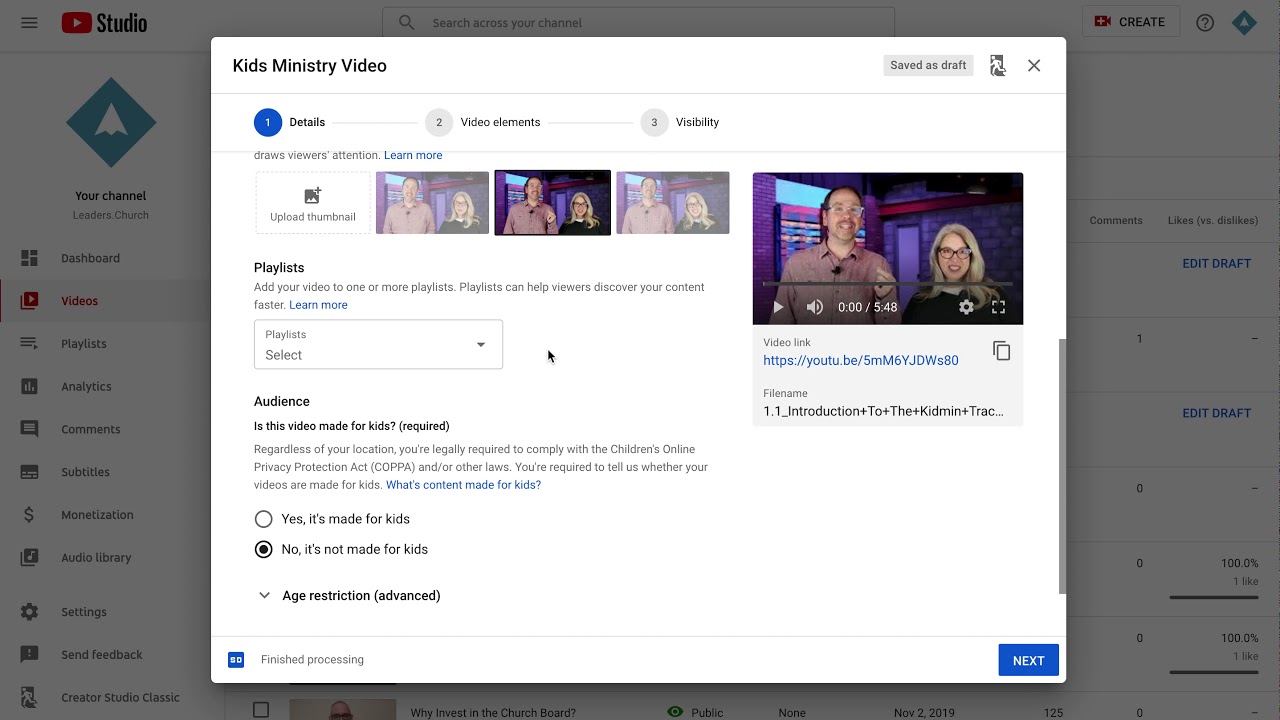This screenshot from YouTube Studio illustrates the detailed layout of the video publishing process. The interface features the familiar, straightforward design with its predominantly white background, intersecting gray lines and segments, accented by YouTube's iconic red elements. The background screen is dimmed to highlight an overlay menu which displays key channel information and navigation links such as Dashboard, Videos, Playlists, and Analytics. 

In the forefront, a white dialog box takes center stage, showcasing the video details interface. The working title, "Kids Ministry Video," is prominently displayed with its current status marked as a draft. To the right, a tiny icon of a person entering a door is positioned next to the typical exit 'X' icon.

This interface is structured as a three-step process: 'Details' (Step 1), 'Video Elements' (Step 2), and 'Visibility' (Step 3). Within the 'Details' section, thumbnail screenshots for the video can be seen, emphasizing their role in viewers' selection. Below, the user is prompted to add the video to one or more playlists, with an informative note on how playlists improve content discovery. A drop-down box for selecting playlists is currently inactive, marked by the placeholder 'Select.'

Further down, the audience designation section asks if the video is made for kids, citing the requirements of the Children’s Online Privacy Protection Act (COPPA). Despite being a kids ministry video, the selection indicates 'No,' it is not made for kids. Finally, a 'Next' button is apparent at the bottom, signaling the ongoing progress in filling out the necessary information for publishing this video.